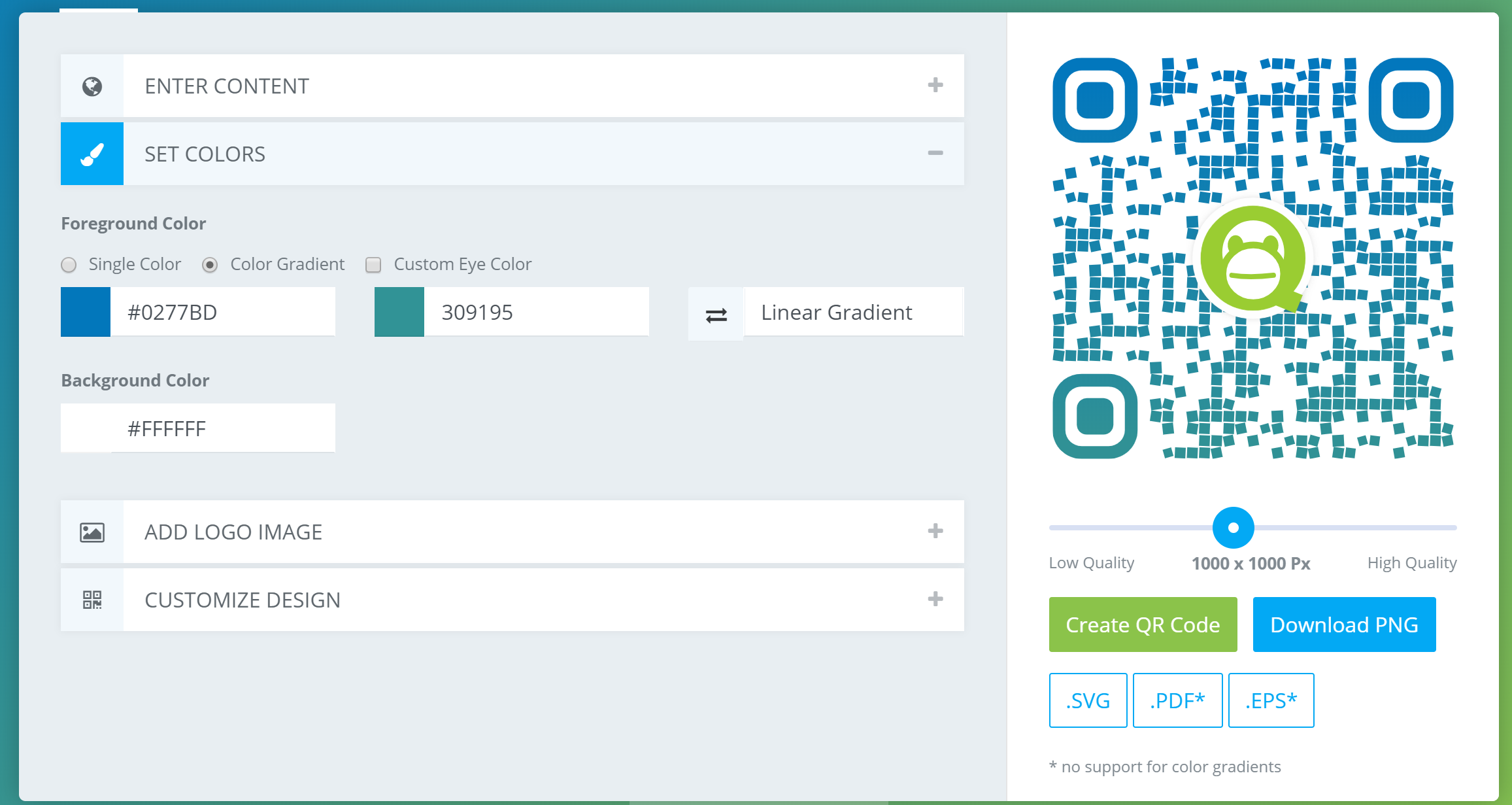The image appears to be a detailed printout of a QR code generator interface. The interface features a clean, white background with some sections highlighted in gray and bordered by various shades of green, giving it a modern and organized look. 

At the top of the interface, there is a row labeled "Enter Content," followed by another row titled "Set Colors." On the left, there's a small square icon depicting a white object against a blue background. Moving down, there are options for "Foreground Color," and within this, selections for "Single Color," "Color Gradient," and "Custom Eye Color." The "Color Gradient" option is currently selected, indicated by a dot.

Next, there are choices for specific gradients, such as "0277BD," "309195," and "Linear Gradient." For the "Background Color," the color code "#FFFFFF" (white) is provided. Below this, there are additional features like "Add Logo Image" and "Add Customized Design."

On the right side of these options, there's a clickable button to choose between low and high quality, along with the number of pixels. The interface allows users to create their own QR code and offers various download formats including PNG, SVG, PDF, and EPS.